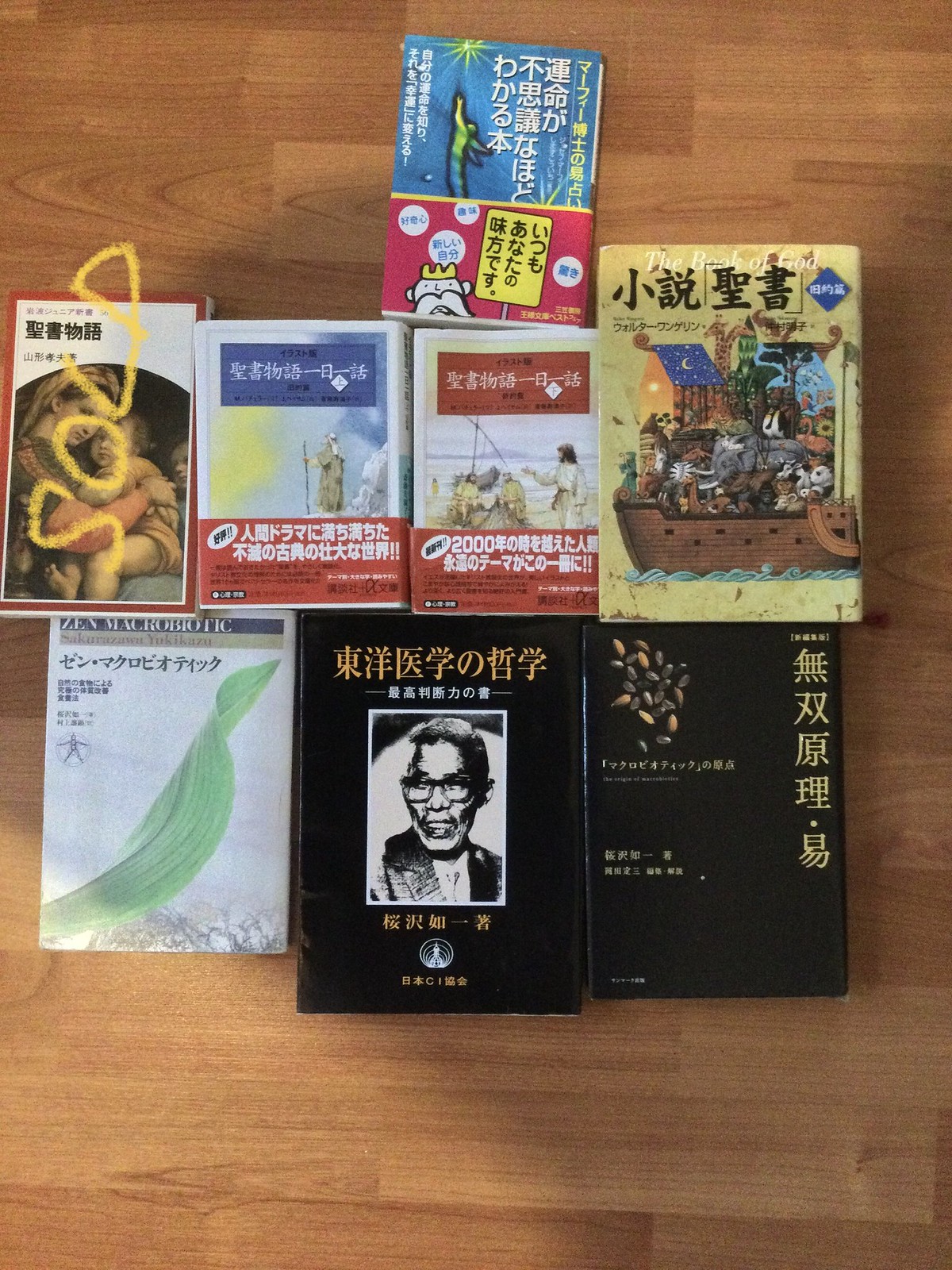This detailed photograph captures a display of eight books arranged neatly on a light brown wooden surface. All the books are in Japanese, and various images and font styles cover their fronts, emphasizing their foreign language. Superimposed in yellow on the left side of the image is the word "sold," indicating that the book in the upper left corner has already been purchased.

The top row features a single book with a distinctive blue and pink cover, depicting a boy with wings reaching for a star, likely aimed at children. The middle row contains four books. The first book on the left in this row appears blue and pink with a drawing of a lady and a baby, and it echoes the "sold" marking. The next two books seem visually connected by their similar themes: one blue and the other red. The last book in this row portrays Noah's Ark, complete with a boat packed with animals and a striking blue flag with a yellow crescent moon.

The bottom row consists of three books. The leftmost book showcases a serene green leaf set against a lighter background. The central book features a photo of Nelson Mandela, identifiable by his iconic features. The final book on the right displays a black cover with an image of a Japanese man wearing glasses, looking to the left, along with some beans in the corner.

Together, these elements reflect a rich diversity of themes and styles, bound by the common thread of Japanese script and cultural imagery.